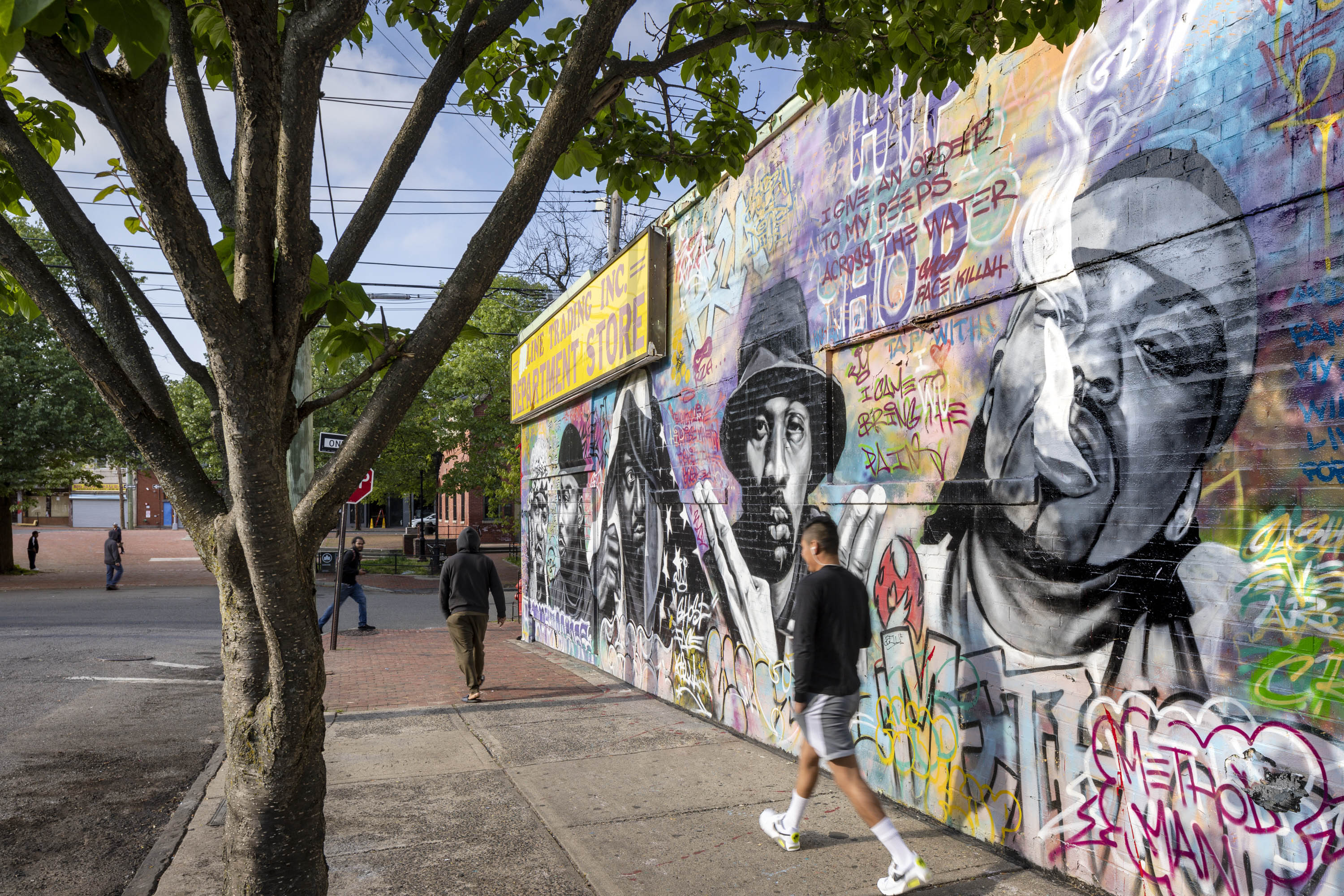This color daytime photograph captures a bustling urban street scene viewed from a sidewalk looking toward an intersection. Dominating the left side of the image is a tree with a trunk and branches extending in a V pattern, adorned with green leaves at the top. On the far left, part of the street moves forward parallel to the sidewalk. 

In the foreground, two men in shorts and black shirts are walking away from us on the sidewalk, heading toward the intersection marked by a stop sign and a one-way sign. Additional men are visible in the distance, walking across the street.

On the right side of the image, the exterior wall of what appears to be a trading ink department store or possibly a liquor store is vividly decorated with street art. This art prominently features faces of African American men, depicted in various styles—one is smoking, with smoke visibly emanating, and another sports a short-brimmed hat. The mural is interlaced with multicolored graffiti, including shades of yellows, reds, blacks, whites, and pastel colors. The bright sun casts shadows from left to right, adding contrast to the vibrant scene.